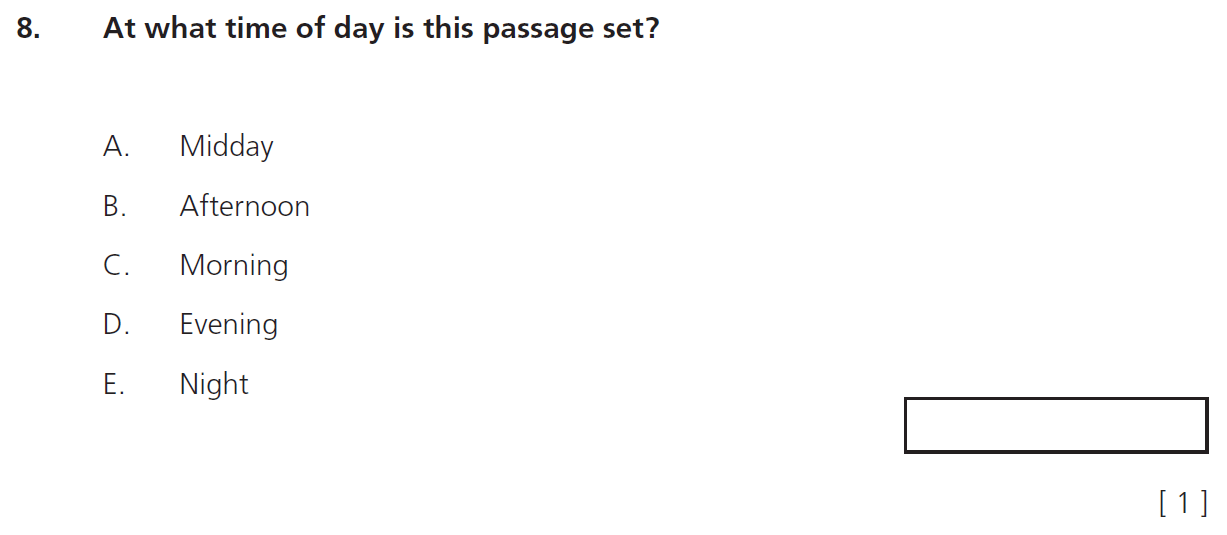In this image, we see a question formatted in a quiz or multiple-choice style, presented on a white background. The question, labeled as "8." in bold black print in the upper left-hand corner, denotes it as the eighth question in a sequence. Following this, the question itself, also in bold black font, asks, "At what time of day is this passage set?"

Below the question, there is a list of potential answers laid out in a bullet-point style, each answer option denoted by a letter from A to E. These options are written in a thinner, gray font compared to the bold question text. The choices are as follows:
- A) Midday
- B) Afternoon
- C) Morning
- D) Evening
- E) Night

In the bottom right-hand corner of the image, there is a rectangular white box with a black border, designed for the user to input their selected answer. Directly beneath this box, there is an additional notation: a pair of brackets surrounding the number "1" ([1]), indicating some form of reference or notation linked to the answer input area.